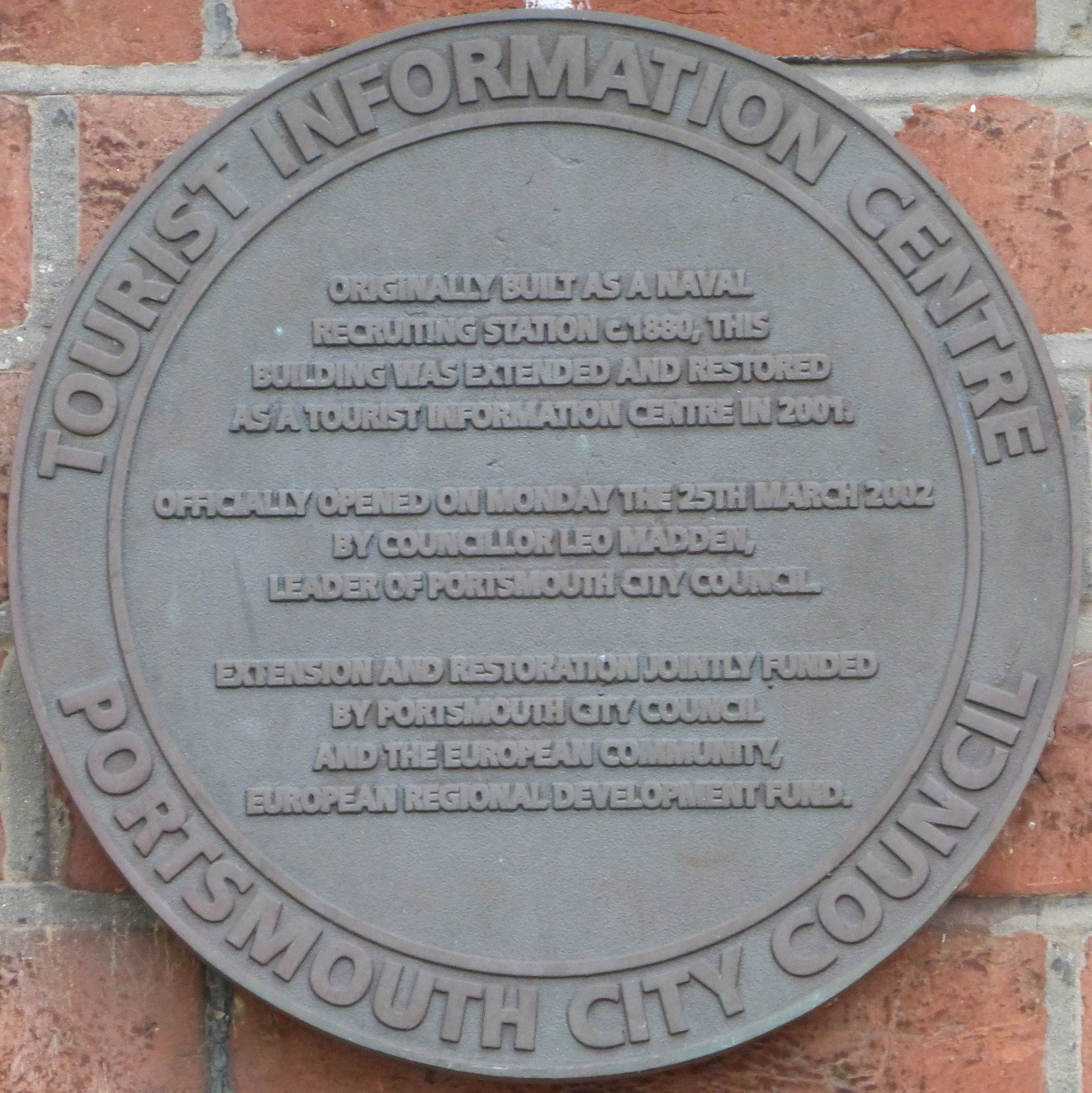The image showcases a close-up of a circular iron plaque mounted on a red brick wall, with the bricks barely visible around the edges. The plaque prominently reads "Tourist Information Centre" at the top and "Portsmouth City Council" at the bottom. The central text explains that the building was originally built as a naval recruiting station around 1880, and later extended and restored as a Tourist Information Centre in 2001. The plaque details that the centre was officially opened on Monday, the 25th of March, 2002, by Councilor Leo Madden, the leader of Portsmouth City Council. Additionally, it notes that the extension and restoration were jointly funded by Portsmouth City Council and the European Community through the European Regional Development Fund. The letters on this silver or grayish metal plaque are raised, adding a tactile dimension to the historical information it conveys.